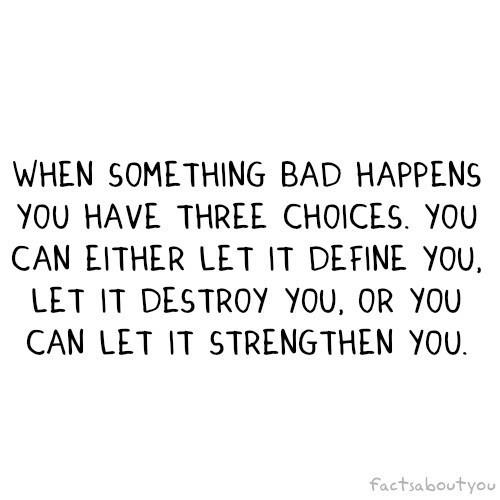The image features an inspirational quote displayed on a stark white background. The quote, written in thin, black, all-caps lettering, spans five lines. The text reads: "WHEN SOMETHING BAD HAPPENS" on the first line, "YOU HAVE THREE CHOICES" on the second, "YOU CAN EITHER LET IT DEFINE YOU," on the third, "LET IT DESTROY YOU OR YOU" on the fourth, and "CAN LET IT STRENGTHEN YOU" on the fifth. In the lower right corner, in a light gray, all-lowercase font, the words "factsaboutyou" are printed without spaces between them. The overall design gives the appearance of a handwritten message on a computer.